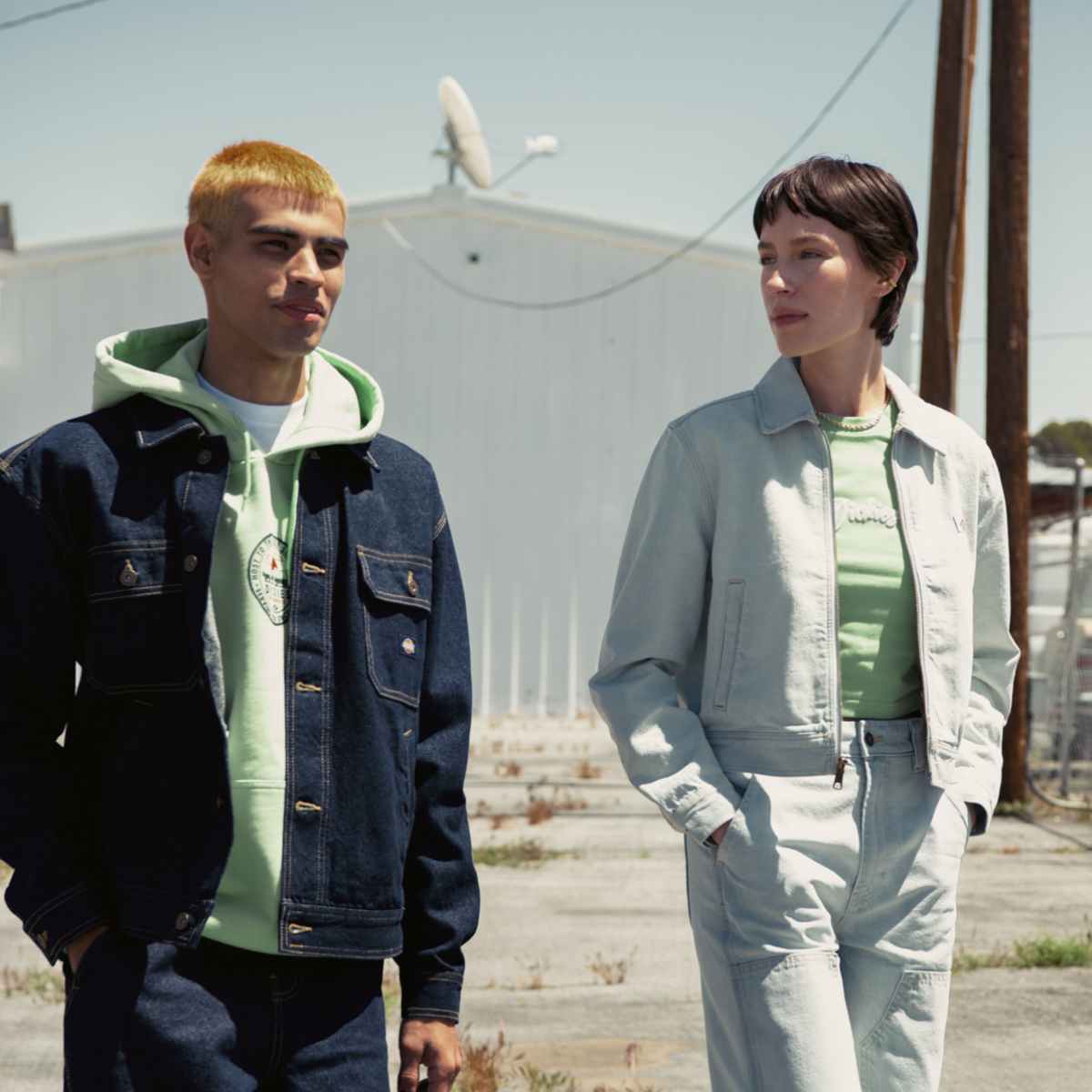The photograph, taken on a bright and sunny day, captures two people walking outdoors on an old cement pavement with grass cropping up through the cracks. On the left is a man with golden blonde hair and black eyebrows, wearing a denim blue jacket, blue jeans, a pastel green hooded sweater, and a white shirt underneath. He has one hand in his pocket. On the right is a woman with short brown hair in a pixie cut, wearing a light blue denim jacket, denim jeans, and a pastel green shirt, accessorized with a necklace. Her hands are also in her pockets, and she is looking at the man. In the background, there is a white building with a dish antenna on top and two tall wooden poles.